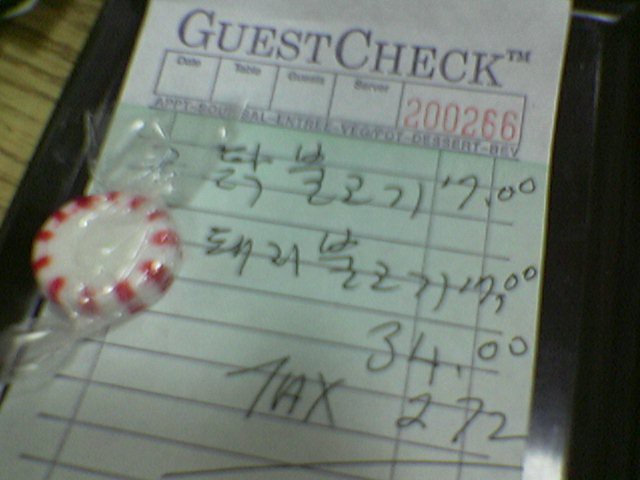A crisp, detailed image showcases a guest check resting on a small black plastic tray. The guest check is predominantly white at the top, printed with blue ink from a register. The header reads "Guest Check TM," followed by structured blocks for details such as date, table, and server, with the number 200266 printed in one of the unlabelled boxes. Below this, the green-lined section indicates the ordered items, listing two separate $17 items amounting to a subtotal of $34 with an additional tax of $2.77. Resting on the left side of the tray is a cellophane-wrapped red and white peppermint candy, adding a finishing touch to the scene.